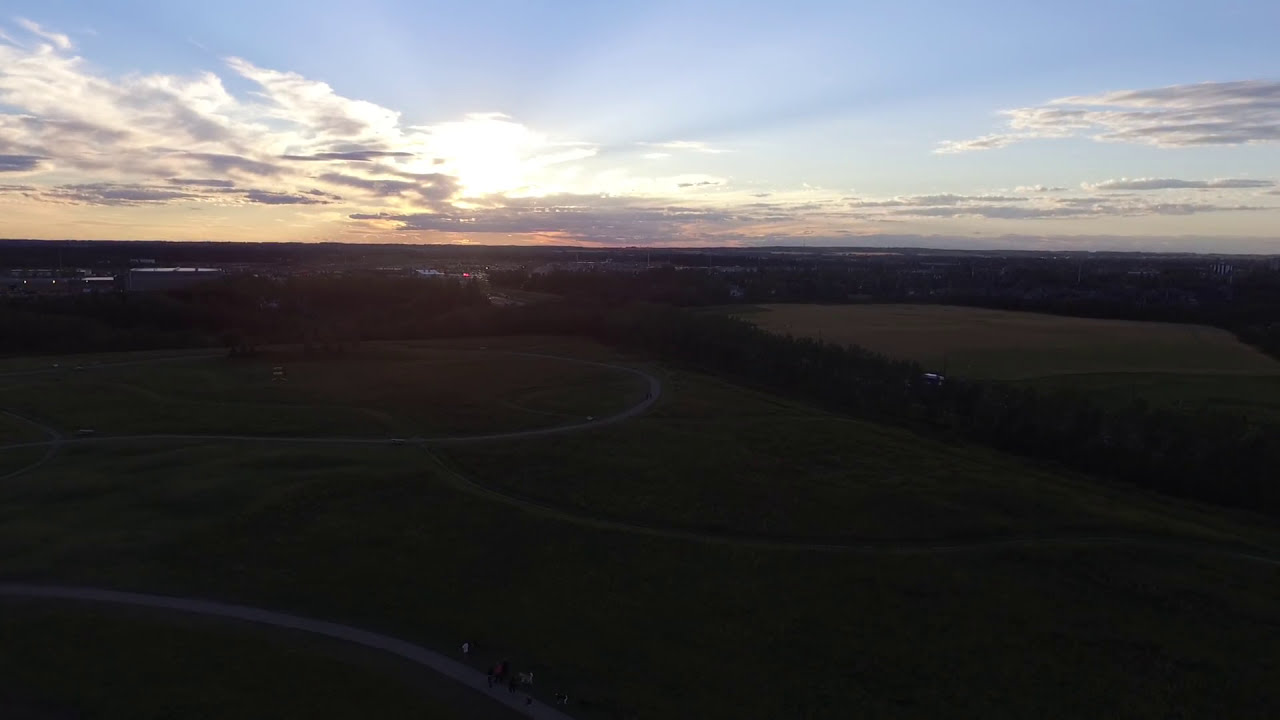The aerial photograph captures a twilight scene, showcasing an expansive grassy field with several pathways meandering through it. The sun is partially obscured by clouds, creating a dramatic interplay of soft yellows, blues, and grays in the sky, suggesting either dawn or dusk. In the lower portion of the image, there are distinct walkways that intersect the grassy terrain, leading towards and away from a cluster of mature trees that diagonally bisect the field. To the right, the landscape transitions into flat farmland with additional trees dotting the horizon. The upper third of the image is dominated by a serene sky, featuring a striking view of scattered clouds illuminated by the rising or setting sun. The overall composition conveys a tranquil, outdoor setting, possibly a park or golf course, enhanced by the subtle presence of people on the walkways and the hint of an urban landscape in the distance.